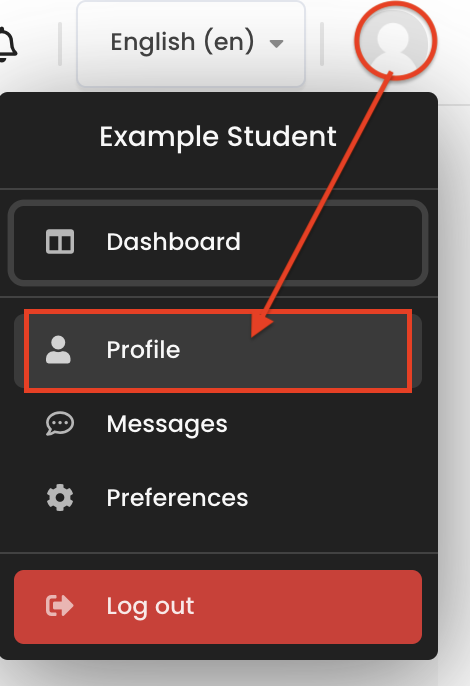This screenshot appears to be a cropped image from either a mobile device, tablet, or desktop, showing a user interface designed for a school-based profile or application setup. 

In the top left corner, there is a black-outlined bell icon set against a gray background, indicative of notifications. Next to it is the text "English EN" with a dropdown menu, suggesting language settings. Adjacent to this, there is a generic profile picture icon, represented by a head silhouette, encircled in red, with an arrow pointing downward to highlight additional details below.

Below this top section, set against a black background with white text, is a list of menu options. The first labeled "Example Student" indicates the user's name. Below it, several icons and corresponding labels are displayed in a vertical alignment:

1. **Dashboard** - symbolized by a window icon.
2. **Profile** - indicated by a head silhouette icon, matching the one encircled in red and pointed to by the red arrow.
3. **Messages** - represented by a chat bubble icon with three dots.
4. **Preferences** - marked by a cogwheel icon.

At the very bottom of the menu, there is a distinct red rectangle with white text and an icon depicting an arrow emerging from a box, labeled "Log Out." This final element indicates the option to log out of the profile or application.

The arrangement and labeling suggest a user interface designed for managing and navigating a school-related profile or application, providing easy access to key features and settings.